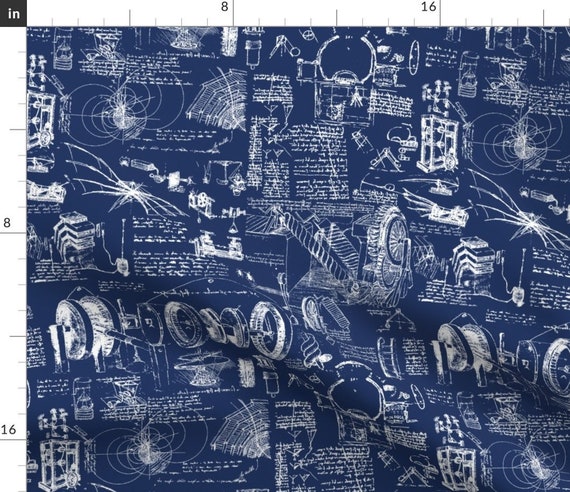The image showcases a square piece of dark navy blue fabric decorated with intricate white prints resembling Leonardo da Vinci's mechanical drawings. The detailed design includes various contraptions and inventions, reminiscent of entries from Da Vinci's notebooks, complete with what appears to be his handwritten notes and schematics, like wheels, square boxes, and other devices. The fabric is slightly wrinkled, confirming its textile nature rather than paper. The layout also features prominent measurement markings: at the top left corner, a black box with the word "inches" in white lettering, and to its right, ruler lines indicating 8 and 16 inches. Similar ruler markings run down the left side of the image, aiding in measuring the fabric. This close-up image emphasizes not only the meticulous Da Vinci-inspired designs but also the practical application of measuring fabric for pattern creation.